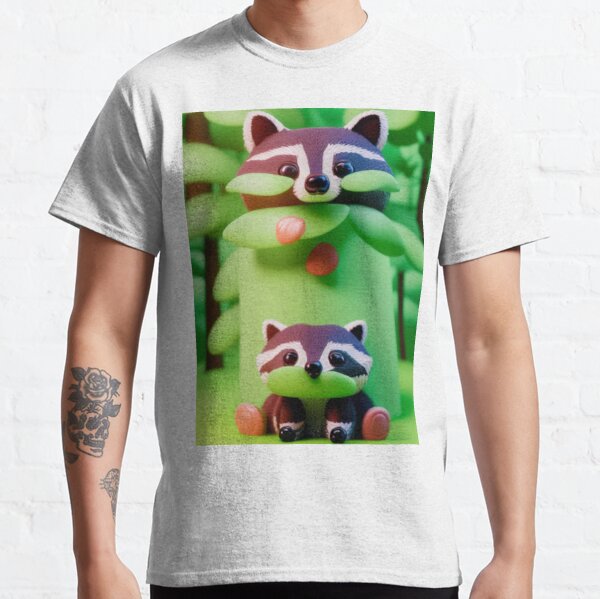This image features the torso of a Caucasian male model against a white background, with the focus primarily on his t-shirt. The man's head is cropped out, and his hands rest by his sides, revealing only his torso from the neck down to the waist. He is wearing dark pants and a white t-shirt, adorned with a prominent rectangular print in the center. This rectangular print depicts a stylized, cartoonish illustration of raccoons. The illustration has a green background with a raccoon peeping out from the top, looking down at a baby raccoon sitting at the bottom with its two front paws and back legs open. The details suggest the raccoons are drawn with brown faces, white trimmings around their ears, and dark eyes, and the top raccoon appears to be hiding behind or standing in a green cup-like object. Notably, the model has a tattoo on his right forearm, positioned on the left side of the image.